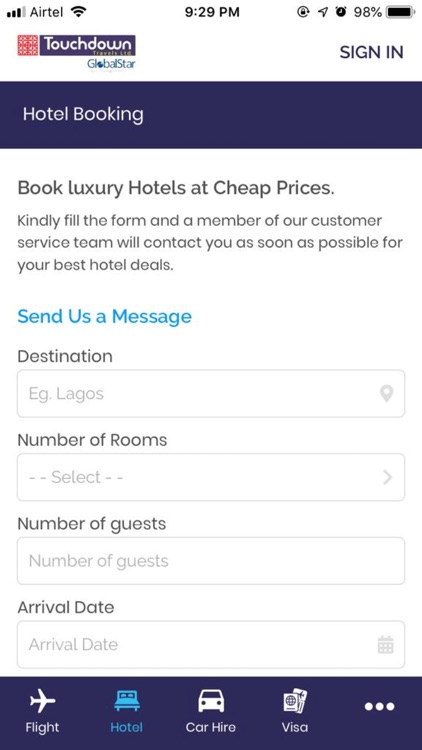The image is a screenshot from a smartphone with a white background. At the top left corner, the mobile carrier "Airtel" is displayed in black, alongside the Wi-Fi signal icon. The time, "9:29," is shown prominently in the center, while the battery icon on the top right indicates a 98% charge.

On the website displayed, the top left corner features the word "Touchdown" in white text against a dark purple rectangular background. Adjacent to it is a red square with a geometric design comprising four smaller squares within it. Below "Touchdown," the words "Global Star" appear in blue on a white background. 

A thick, dark purple line runs across the screen beneath this, with the phrase "Hotel Booking" in white font centered on it. Underneath this section, also on a white background, is a headline in light gray reading, "Book luxury hotels at cheap prices." The headline is followed by a note instructing users to fill out a form for contact from customer service regarding the best hotel deals.

Further down, the form fields are visible, allowing users to enter details such as the destination, the number of rooms, the number of guests, and the arrival date.